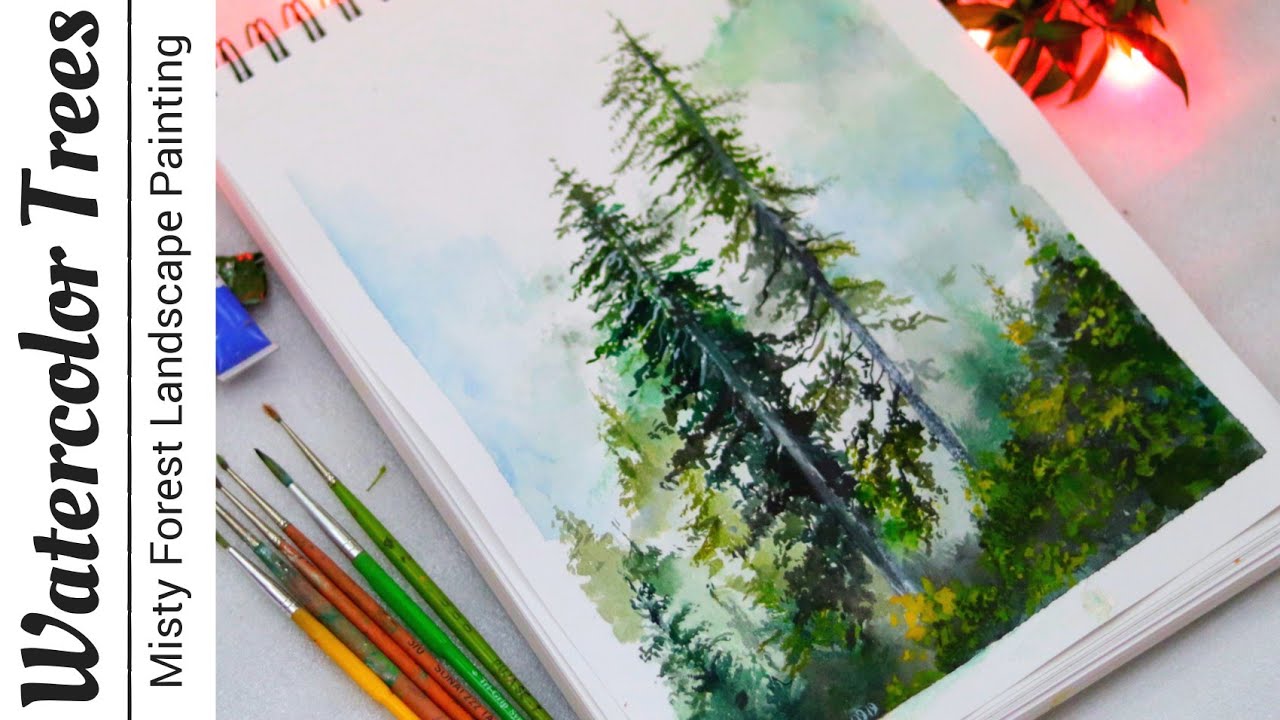The image depicts a small notepad with a watercolor painting of a misty forest scene, featuring various evergreen trees and dense shrubs. The pad, edged with white and light blue, is positioned centrally, showcasing the detailed nature artwork. To its left lies an assortment of art supplies: six paintbrushes with colorful handles—two green, two red, one brown and green, and one yellow—positioned below two visible tubes of paint, one cobalt blue and the other likely black. In the top right corner, a red flower peeks into the frame. The left side of the image is marked by vertical black text on a white background, reading from bottom to top: "Watercolor Trees, Misty Forest, Landscape Painting." The composition suggests either an advertisement for a watercolor class or a showcase of the artist's work.